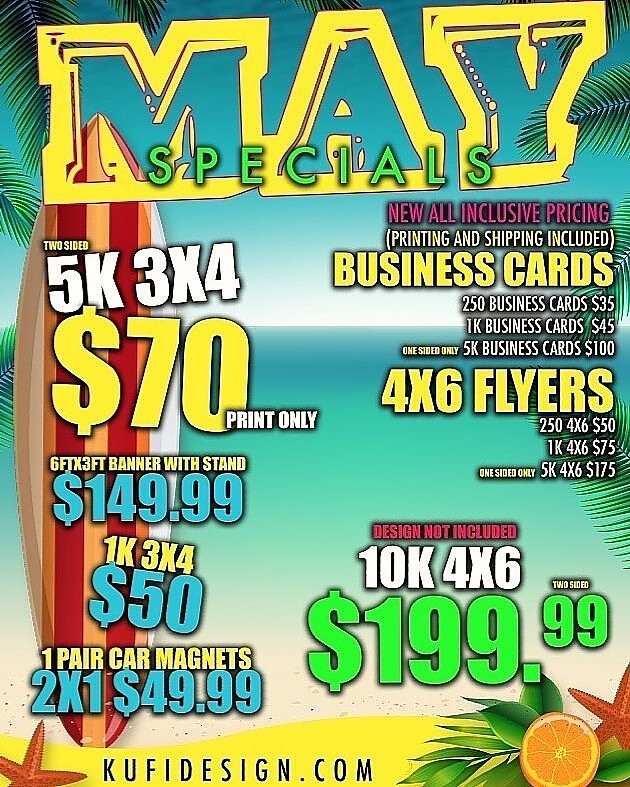The image appears to be a vibrant advertisement poster, prominently featuring a tropical-themed background rendered in digital art. The serene beach scene includes details such as sand at the bottom, transitioning teal to dark blue-green waters, and palm leaves encroaching from the sides. A vertically standing surfboard, striped in brown, red, orange, and white, occupies the left side of the image. The poster is headlined with "May Specials" in large blue text bordered by yellow, capturing attention with its eye-catching design reminiscent of a magazine cover.

Throughout the poster, various promotional offerings are advertised in vivid colors. Positioned on the right side in red text, "New All-Inclusive Pricing" is highlighted, followed by the white text in parentheses, "Printing and Shipping Included." Below this, the deals are listed: "Business Cards" in yellow text with specific offers such as "$250 Business Cards, $35," "$1K Business Cards, $45," and "$5K Business Cards, $100."

On the left side, more deals are presented, including "One-Sided Only" in yellow, followed by "4x6 Flyers," also in yellow, with pricing details like "$250 4x6, $50" and "$1K 4x6, $75." Additional promotional items feature "5K 3x4 for $70," "a gift banner with a stand for $149," and "a pair of car magnets, 2x1, $50." At the bottom, the image includes text for a website, reinforcing the retail branding.

Overall, the poster exudes a colorful, beachy ambiance while detailing numerous print and shipping offers available during the May Specials.